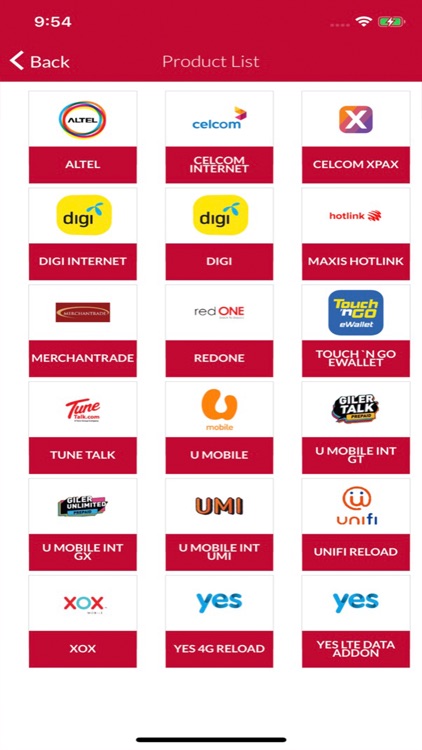The image displays a comprehensive product list featuring logos from 18 different companies. The companies included in the list are Altel, Silcom, Silcom X-Pax, Digi Internet, Digi, Maxis Hotlink, Merchantrade, RedOne, Touch 'n Go Wallet, TuneTalk, U-Mobile, U-Mobile INTGT, U-Mobile INTGX, U-Mobile INTUMI, UNIFI Reload, XLX, YES 4G Reload, and YES LTE Data Add-On. 

At the top of the image, a banner resembling a mobile or cell phone interface shows the time as 9:54. To the right of the time, there are small, unreadable letters followed by icons indicating full Wi-Fi signal strength and a fully charged battery.

Below the banner, an interface signal with a "back" button is present, allowing users to navigate back to the previous screen. Following this, the product list is displayed. Each product is showcased within a dual-colored rectangle, where the top two-thirds is white and the bottom third is red. The company's name is written in white letters within the red section, and their respective logos are situated in the white portion.

Detailing each logo:
1. Altel: A red and blue circle containing the company name.
2. Silcom: Red text with a red symbol above it.
3. Silcom X-Pax: Red colored with a white "X".
4. Digi Internet: Yellow background resembling a leaf with "Digi" written in black.
5. Digi: Same as Digi Internet with the yellow leaf background.
6. Maxis Hotlink: Red text with an accompanying red logo.
7. Merchantrade: Features a red background with white text that is difficult to read.
8. RedOne: The name split into "Red" in blue letters and "One" in red letters on a white background.
9. Touch 'n Go Wallet: Blue background with "Touch 'n Go" in yellow and "E-Wallet" in white below.
10. TuneTalk: Red letters on a white background.
11. U-Mobile: Orange graphic with "Mobile" written below.
12. U-Mobile INTGT: White letters with a yellow icon that is too small to discern clearly, followed by a blue talk signal.
13. U-Mobile INTGX: Similar to U-Mobile INTGT but specific lettering is not readable.
14. U-Mobile INTUMI: The letters "UMI" appear in a 3D style.
15. UNIFI Reload: The "U" looks like an "at" symbol integrated with a smiley face, followed by "UNI" in red and "FI" in blue.
16. XLX: An "X" is red, "L" is blue, and the next "X" is red.
17. YES 4G Reload: Blue text.
18. YES LTE Data Add-On: Blue text.

This product list, with its detailed presentation of logos and corporate identities, is organized to provide clear visibility and easy recognition of each company.